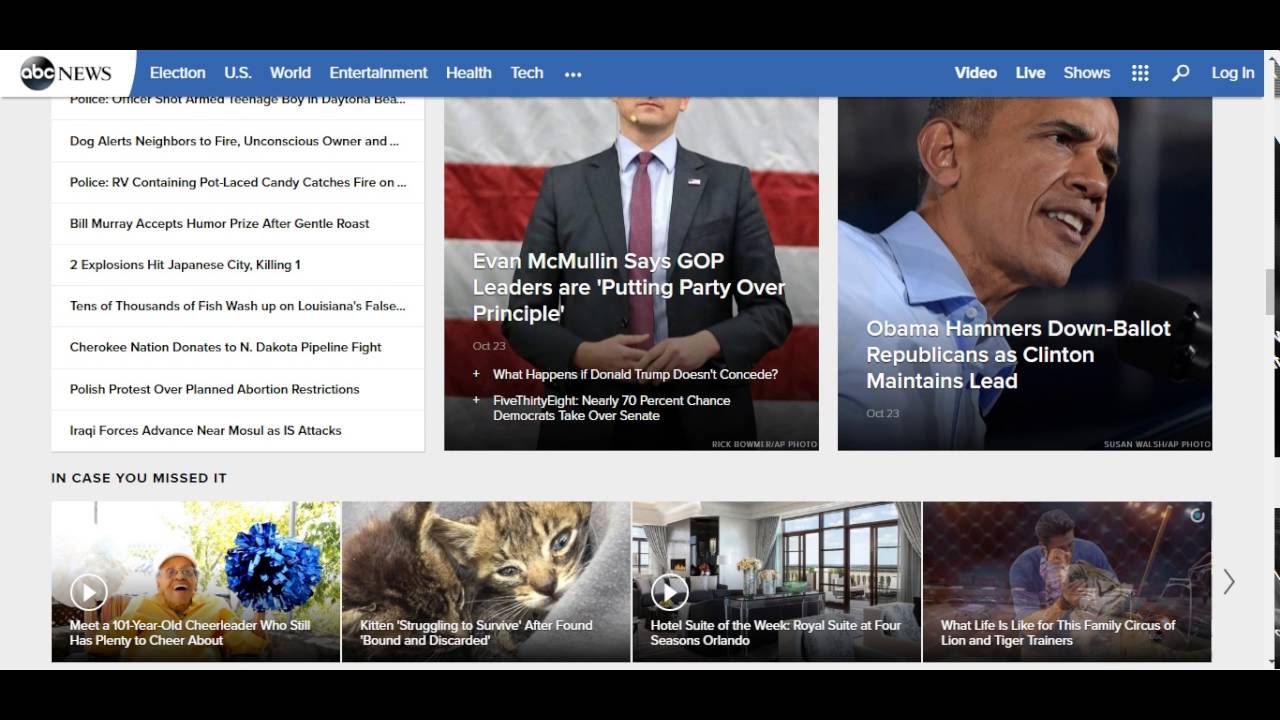In the image, there is a blue header, adorned with white tabs starting from the top left. The header begins with the logo "ABC News", where "ABC" is written in white against a black background, and "News" is in black. The tabs, set against the blue background, read: Election, US, World, Entertainment, Health, Tech, Video, Live, Shows, with Login and Search Party on the far right, all in white text.

Below the header, on the right side of the image, are several news headlines. Prominently featured is a picture of Barack Obama in a blue shirt, accompanied by the text: "Obama Hammers Down Ballot Republicans as Clinton Maintains Lead, October 23." Adjacent to this, still on the right but center-aligned, is the headline: "Evan McMullin Says GOP Leaders Are Putting Party Over Principle, October 23." Below that are additional headlines: "What Happens If Donald Trump Doesn't Concede, 538," and "Nearly 70% Chance of Democratic Takeover in Senate."

On the left side, there are multiple headlines stacked vertically: 
- "Dog Alerts Neighbors To Fire, Police RV Containing Pot-Laced Candy Catches Fire"
- "Bill Murray Accepts Human Rights Crisis After Gently Roasted"
- "Swiss Plushie In Hit Japanese City Killing One"
- "Tens Of Thousands Of Fish Wash Up On Louisiana's Cherokee National Donation To End Dakota Pipeline Fight"
- "Polish Protest Over Planned Abortion Restriction"
- "Iraqi Forces Advance Near Mosul, ISIS Attacks"

At the bottom of the image, under the section titled "In Case You Missed It," starting from the left, are more stories:
- "Meet A Year-Old Cheerleader Who Still Has Plenty To Cheer About"
- "Kitten Struggling To Survive After Being Found Bound And Discarded"
- "Hotel Suite Of The Week, Royal Suite At Forces In Orlando"
- "What Life Is Like For The Family Circus Of Lion And Tiger Trainers"